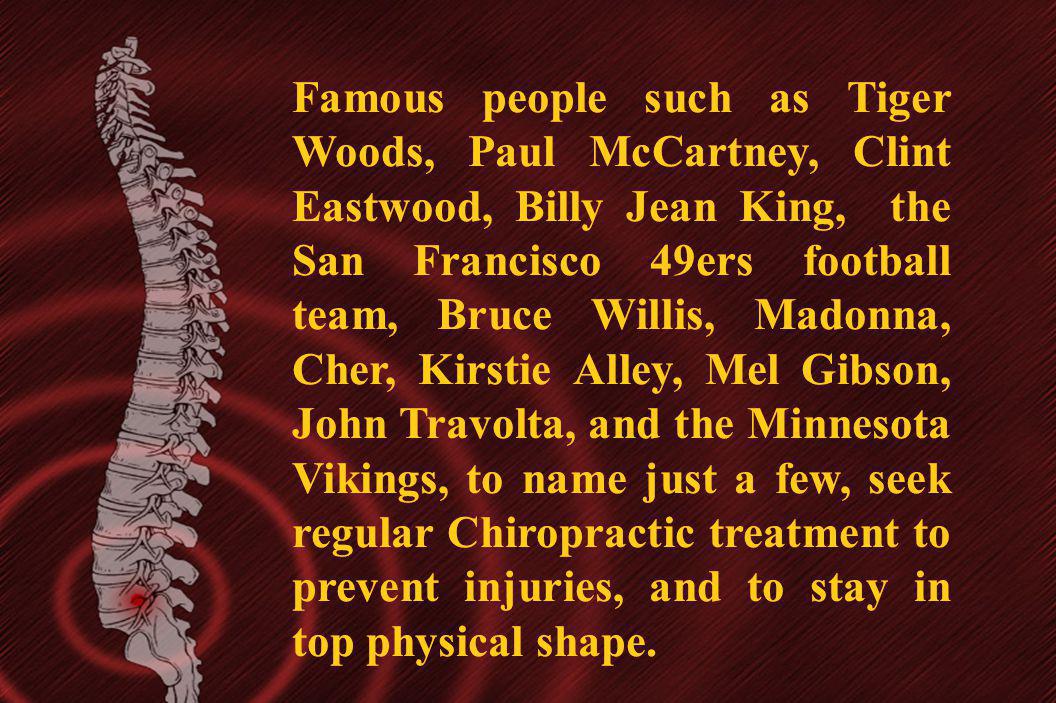This image features a striking dark red, textured background with a prominent visual of a human spine on the left-hand side. The spine is depicted in a light grey color, showcasing the intricate details of the vertebrae. At the very bottom of the spine, there is a vivid red spot, from which light red concentric circles emanate outward, giving the appearance of ripples spreading across the image. To the right of the spine, in a yellow serif font, the text reads: "Famous people such as Tiger Woods, Paul McCartney, Clint Eastwood, Billie Jean King, the San Francisco 49ers football team, Bruce Willis, Madonna, Cher, Kirstie Alley, Mel Gibson, John Travolta, and the Minnesota Vikings, to name just a few, seek regular chiropractic treatment to prevent injuries and to stay in top physical shape." The text is aligned centrally with a one-inch margin surrounding it.